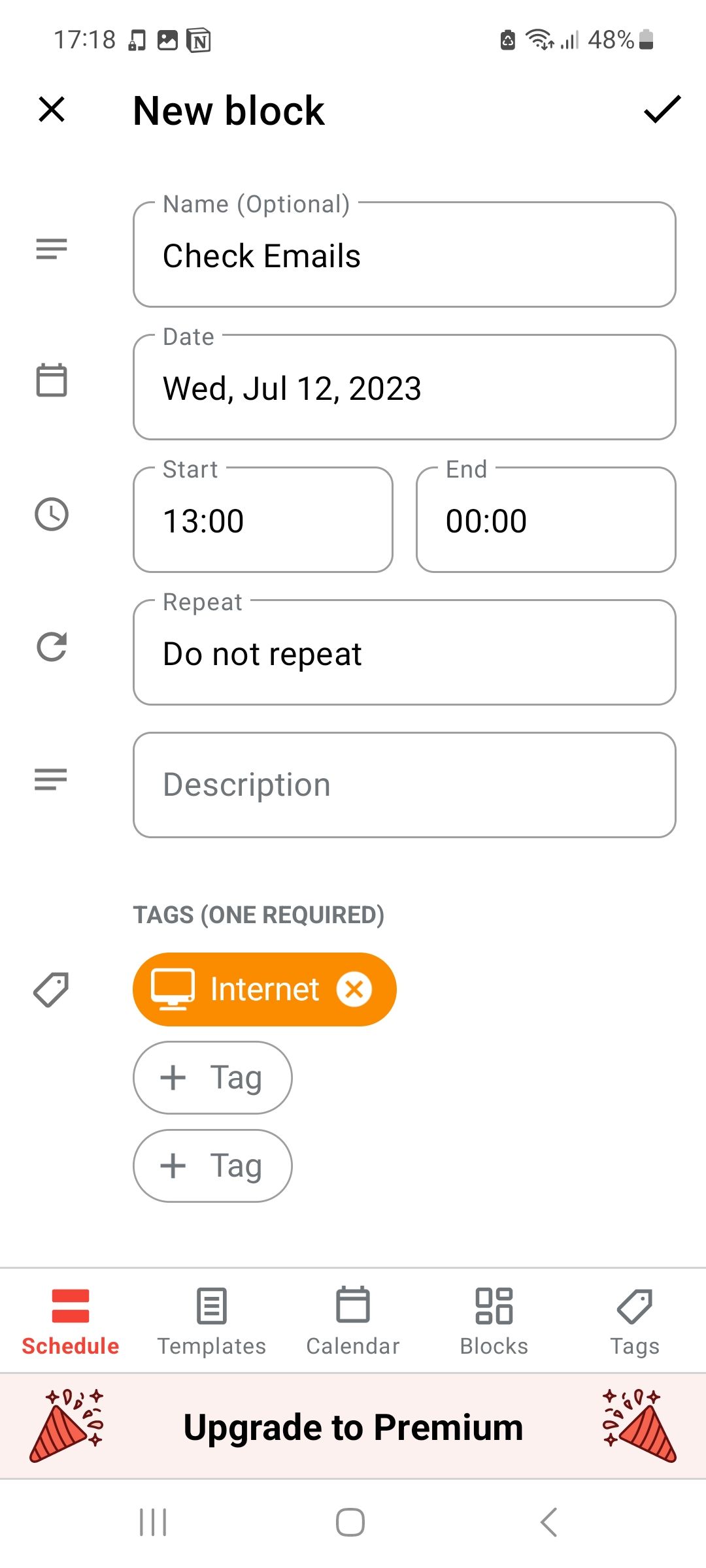The image appears to be a screenshot taken on a smartphone, displaying a work-related website or application. At the top right of the image, there is a vertical battery indicator, showing it is about half full, with "48%" written next to it. To the left of the battery, there is a signal strength icon with three out of four bars filled, followed by a Wi-Fi signal strength icon with all four bars filled. On the top left corner of the screen, the current time is displayed in military format as "17:18".

Adjacent to the time, there are several small icons: a phone icon with a lock symbol at the bottom left, a photo icon, and a block icon with the letter "N" on it. Below this top section, in bold black font, are the words "New Block." On the left side of "New Block" is an "X" symbol, and on the far right of it is a check mark symbol.

Below these headings, the screen is divided into several rectangular boxes. The top rectangular box is labeled "Name." The box immediately below it is labeled "Date." There are two smaller rectangles in the middle, labeled "Start" and "End." The next set of two boxes is labeled "Repeat," and the last box at the bottom does not have any label on its outer side.